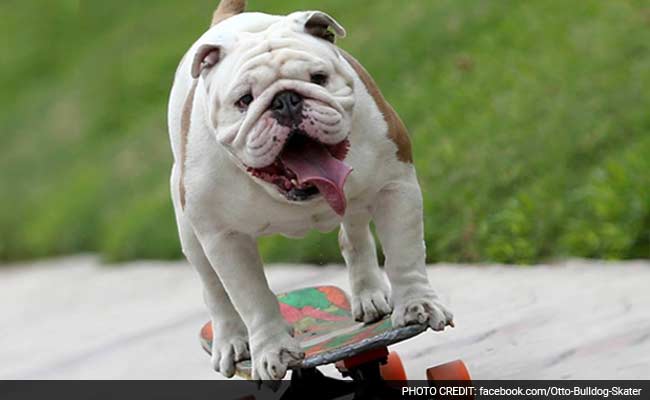In this outdoor image, a chubby, white bulldog with brown patches is captured riding a skateboard on a slightly blurry gray sidewalk. His long pink tongue hangs out as he pants heavily, leaning slightly to the left. The skateboard, with a colorful green, orange, and red design and orange wheels, supports all four of his paws. He looks straight at the camera with his wrinkly face framed by folded ears and a stubby brown tail peeking from behind. The background features a blurred green expanse, possibly grass or foliage. At the bottom right corner, a credit reads "photo credit: facebook.com/otto-bulldog-skater" in all caps against a thin, dark gray border.